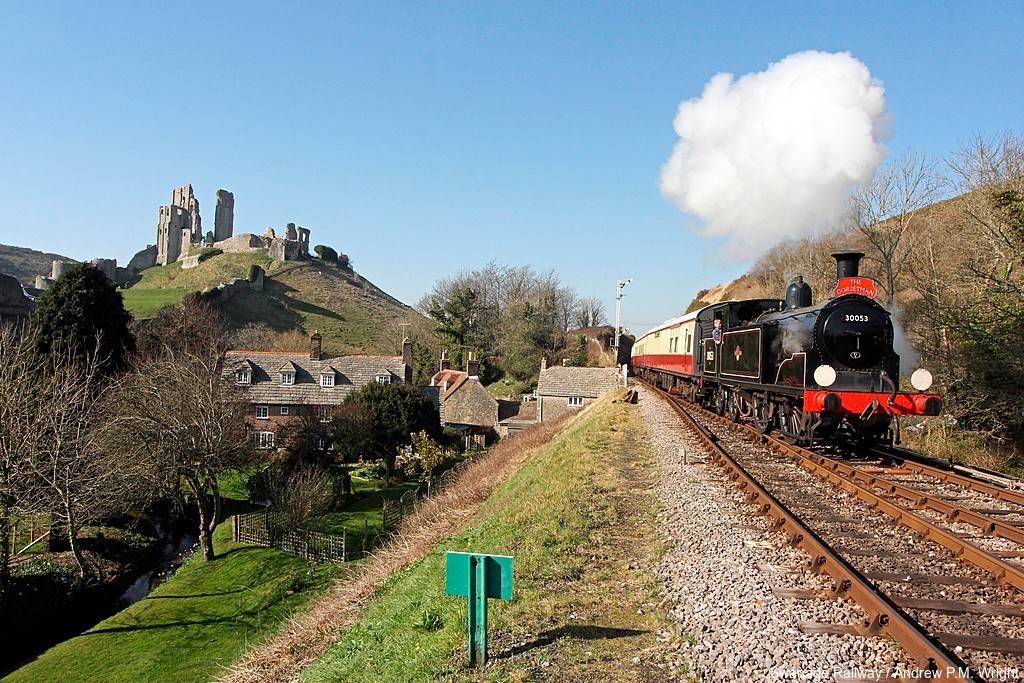The photograph captures a dynamic scene of a steam locomotive chugging towards the viewer from the right side, its white smoke billowing from the chimney. The black engine, accented with a red front bumper and a red nameplate with light tan lettering, leads a short train of two or three cars that are primarily white with red trim along the lower quarter. Traversing a track that veers slightly right and runs parallel to another track to its left, the train is nestled between two hillsides. The right hillside is void of structures, offering a pleasant spot to sit and watch the trains pass by. The hillside to the left has a small hillside at the base with brown and green grass and a green sign in the middle and the backdrop of a large brick home built against the gravel bordering the train tracks. An intriguing feature is the ruins on the left hill’s crest, reminiscent of a castle, adding historical intrigue. A small creek runs from the bottom left corner, winding up and to the right before curving left again. In the far background, atop another hill, possible ruins or a stone structure resemble a Stonehenge-like construct, wrapping the image in ancient mystique. Above it all, a clear blue sky frames the scene, harmonizing with the picturesque landscape of rolling hills and residential buildings.